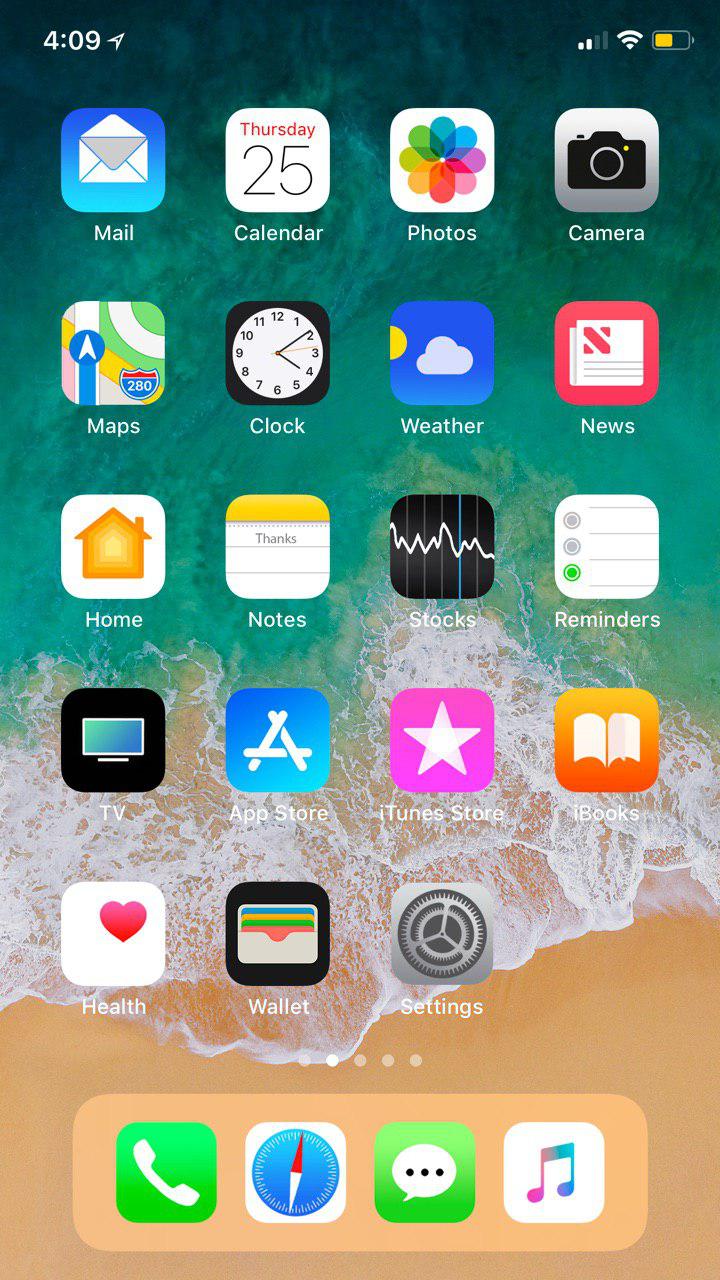This is a detailed screenshot of an Apple iPhone home screen taken at either 4:09 or 9:04 AM, which is indicated by the clock at the top left corner, without specifying "AM" or "PM." On the top right, the battery icon shows a 50% charge. The home screen displays a total of 23 application icons organized into five rows of four apps each and a final row with three apps.

In the first row, from left to right, are the icons for Mail, Calendar, Photos, and Camera. The second row includes Maps, Clock, Weather, and News. The third row features Home, Notes, Stocks, and Reminders. The fourth row contains the TV app, App Store, iTunes Store, and iBooks. The fifth row from the left has Health, Wallet, and Settings.

At the bottom of the screen, there is a navigation bar with four icons: a Phone icon on the far left, followed by a Safari (compass) icon, a Messages icon, and finally the Music app icon on the far right.

The wallpaper in the background captures a serene beach scene with a close-up view: the sandy shore at the bottom transitioning into aquamarine ocean water towards the top.